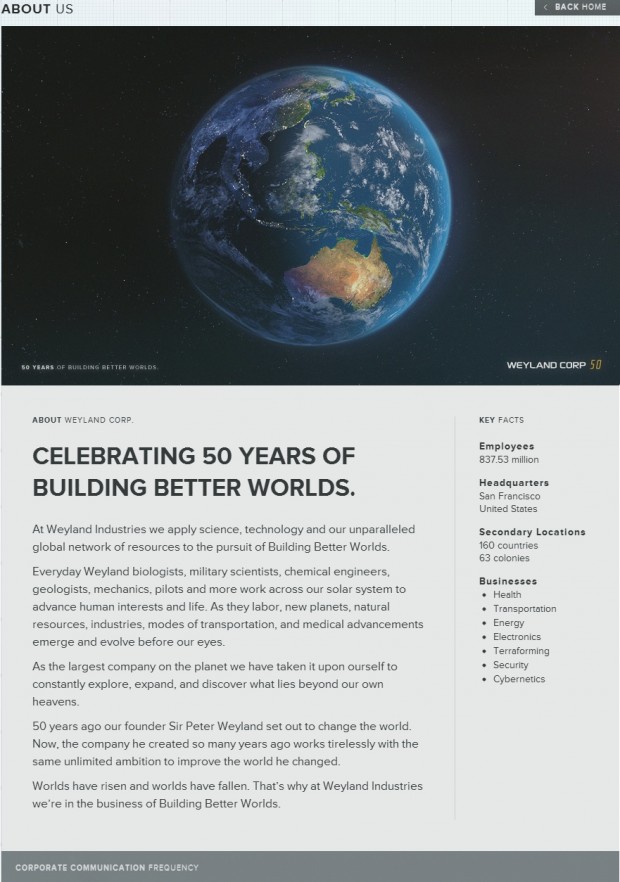The image resembles a page from a magazine, prominently featuring a glossy promotional spread for Weyland Corp. The top third of the image is dominated by a striking black rectangle with a detailed, high-resolution depiction of Earth as seen from space. This view highlights the deep blue of the oceans and the swirling white clouds, with the recognizable brown landmass of Australia visible at the bottom of the globe.

Beneath this captivating image, the rest of the page is dedicated to text celebrating Weyland Corp’s 50-year anniversary. The bold headline reads, "Celebrating 50 Years of Building Better Worlds," followed by a subheading, "About Weyland Corp." This section elaborates on the corporation's mission, stating: "At Weyland Industries, we apply science, technology, and our unparalleled global network of resources to the pursuit of building better worlds." The text continues with several paragraphs praising the company’s achievements and ethos, concluding with, "Worlds have risen and worlds have fallen. That's why at Weyland Industries, we're in the business of building better worlds."

To the right of the main text block, a sidebar titled "Key Facts" provides concise company statistics: "Employees: 837.53 million," "Headquarters: San Francisco," "Secondary Locations in 160 countries and 63 colonies," and a summary of their diverse business sectors, including health, transportation, energy, electronics, terraforming, security, and cybernetics.